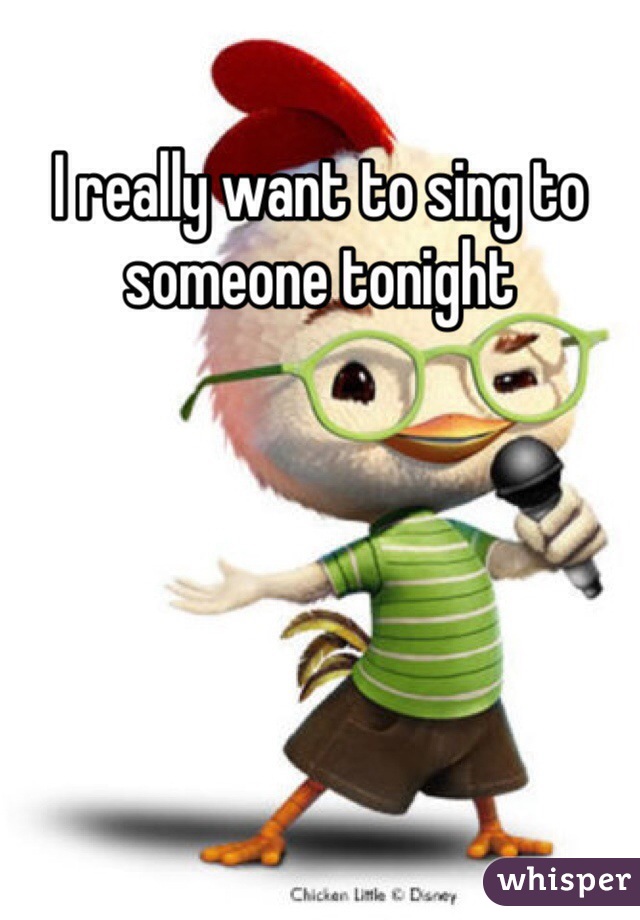This meme features an animated, anthropomorphic character from Disney's "Chicken Little." The central figure is Chicken Little himself, instantly recognizable with his oversized, white-feathered head, expressive black eyes framed by bright green glasses, and a smiling orange beak. He sports two rooster combs on top of his head, further emphasizing his quirky, endearing look. Chicken Little is clad in a light green t-shirt adorned with dark green and white horizontal stripes, paired with dark brown shorts. He holds a microphone in his left wing, suggesting he's ready to belt out a tune. The meme text above reads, "I really want to sing to someone tonight," making it a playful, karaoke-themed image that friends might share for fun. The clean white background emphasizes the character, with "Chicken Little © Disney" in the bottom left corner and a Whisper app logo in the bottom right, adding to the meme's modern, digital age feel.